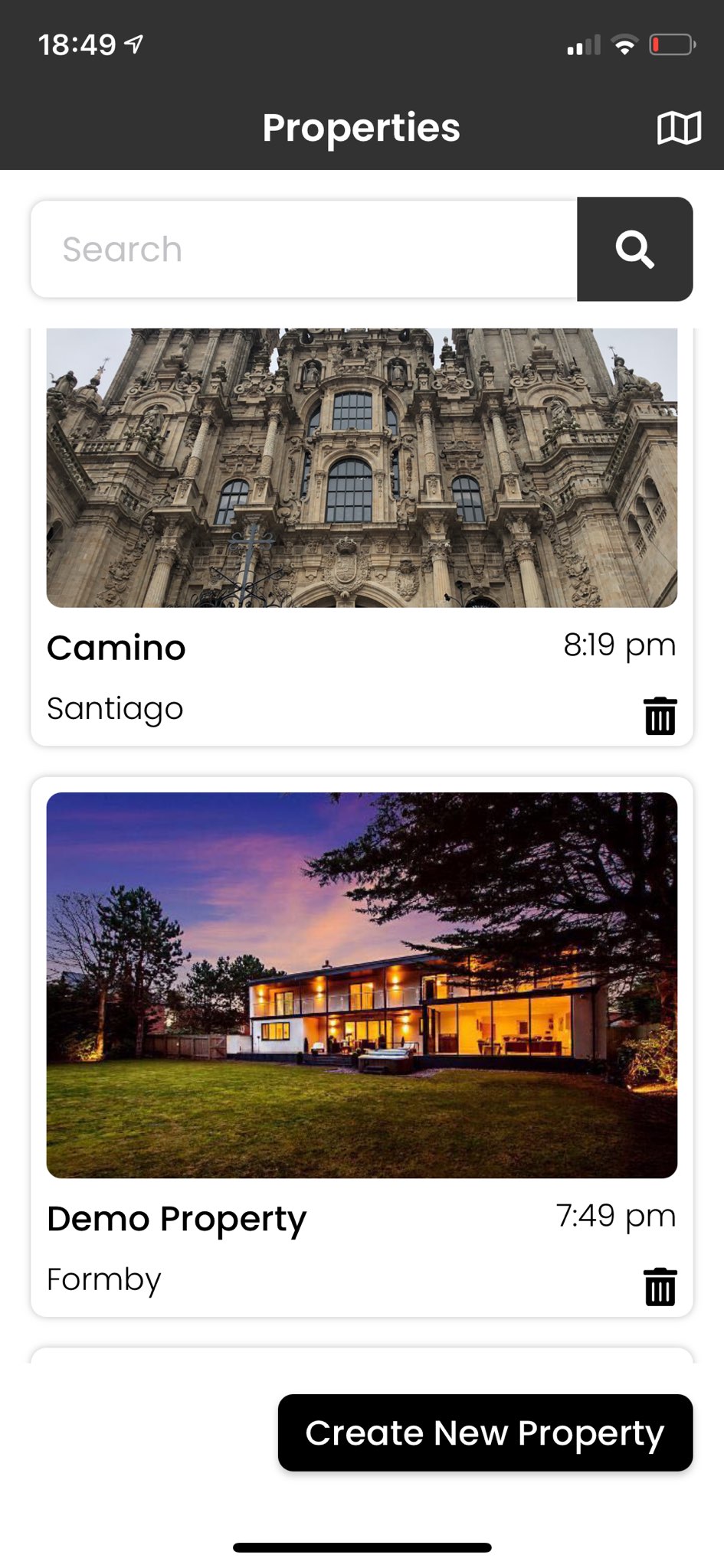The screenshot displays a computer interface with a prominent black bar at the top. On the left side of the bar, the current time is shown in white text. To the right of the time, there's a send arrow, and further to the right are three icons indicating reception, Wi-Fi connectivity, and battery status.

A few lines down, centered in white text, the term "Properties" is displayed alongside a page icon. The background below this section is white, featuring a centered, rectangular search bar outlined in gray. Inside the search bar, the word "Search" appears on the left side in gray text, and on the right, there's a black square with a white magnifying glass icon.

Beneath the search bar is an image of a stone building resembling a church or a college, taken from a low angle. Below this image, on the left side, the word "Camino" is presented in bolded black text, while the time "8:19 PM" is noted on the right in black text. Two lines below, the word "Santiago" is displayed in black text on the left, with a wastebasket icon on the right.

Further down, another image appears, depicting a long, two-story house. Below this image, "Demo Property" is written in bolded black text on the left, with "7:49 PM" in black text on the right. Underneath this, on the left, the text "Form by" is shown in black, accompanied by a trash can icon on the right.

At the bottom right of the screenshot, there is a black button with "Create New Property" written in white text.